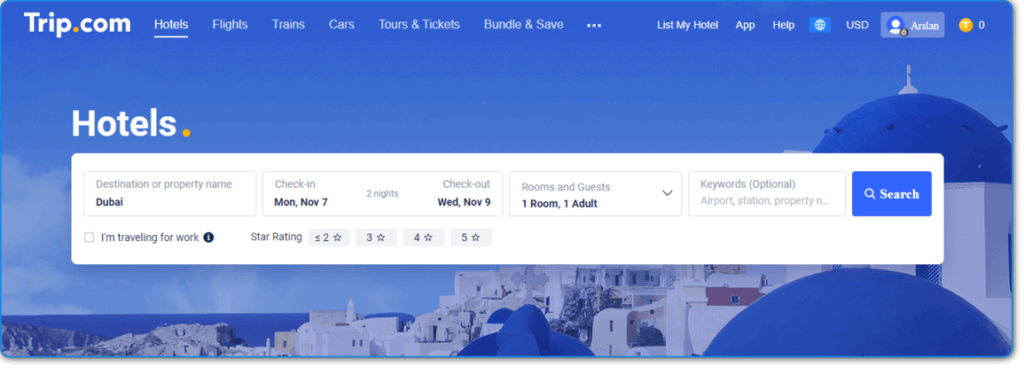This image showcases the Trip.com website, which prominently features a cityscape backdrop. The scene consists of numerous large white buildings and homes perched on hills, all under a partly cloudy blue sky. At the top left corner of the page, the Trip.com logo is displayed in white, with a yellow dot. Moving right across the top menu bar, the site offers options for "Hotels," "Flights," "Trains," "Cars," "Tours & Tickets," "Bundle & Save," "List My Hotel," "App," and "Help." Nearby, there is a globe icon, the currency indicator "USD," and the user's profile name, accompanied by a coin symbol in the upper right corner.

Centrally placed on the page is a prominent "Hotels" section, marked with a yellow circle. Below, there is an input field for entering information such as the destination or property name, check-in and check-out dates, room and guest numbers, and an optional field for keywords. Additionally, users can sort hotel options by star rating and specify if they are traveling for work.